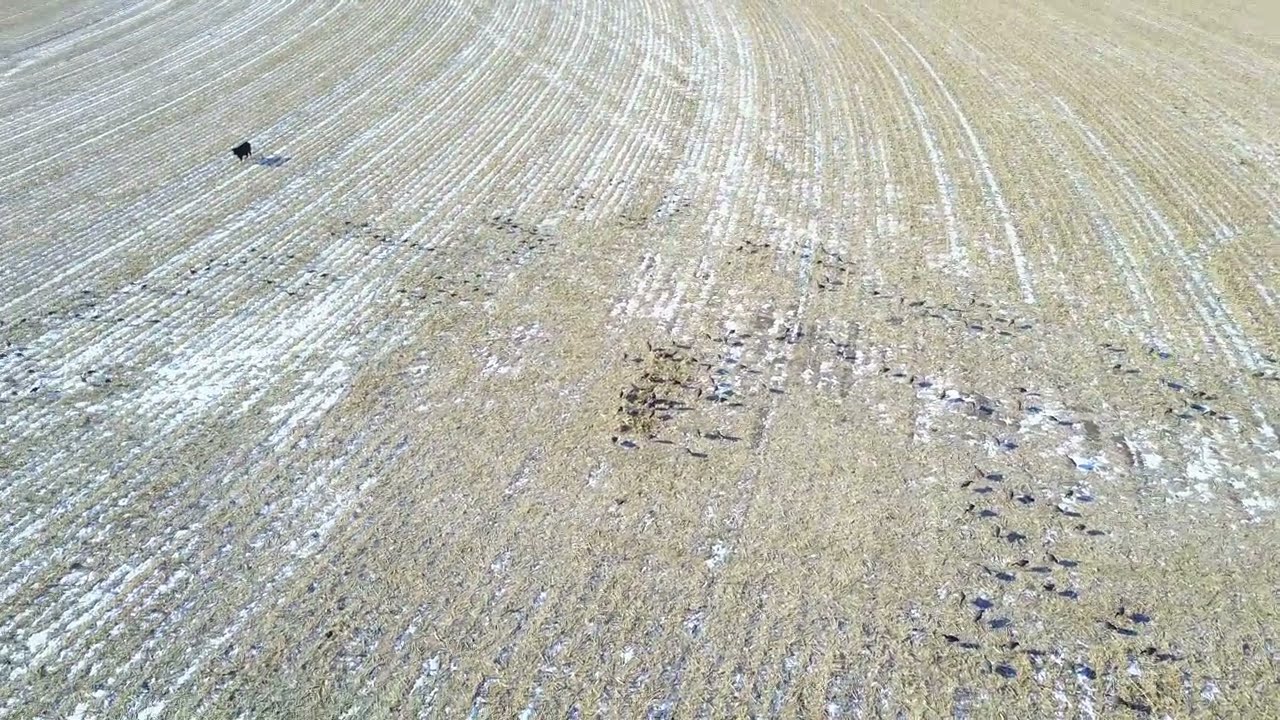This aerial photograph captures a recently harvested field, possibly of corn or wheat, characterized by its tan and beige colors with patches of light-colored dirt and remnants of snow caught in the ridges of the plowed earth. The field features curved, parallel lines, suggesting the work of a tractor. Scattered across the ground, particularly noticeable in the bottom right, are numerous crows, likely feasting on leftover seeds. In stark contrast to the otherwise barren landscape, a single black cow stands in the top left corner, adding an element of curiosity to the scene. The overall image is a blend of natural and agricultural elements, depicting a serene yet slightly odd rural setting.